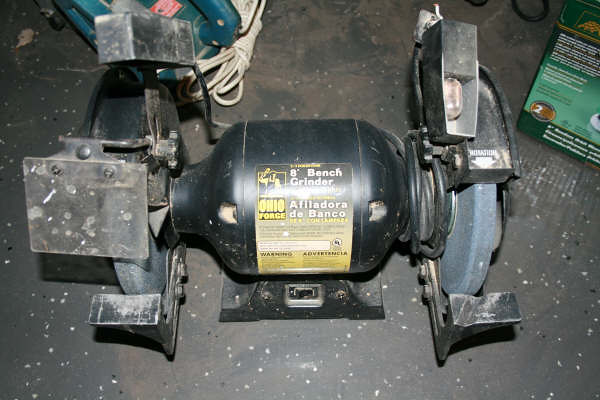This landscape-oriented photograph captures a black bench grinder positioned on a dusty concrete floor. Central to the image is a sticker affixed to the cylinder of the bench grinder. The sticker features the text "8 Inch Bench Grinder," with "afiladora de banco" written underneath in smaller letters. The label displays a mixture of black and yellow outlines, with the primary text in white. Additionally, a logo bearing the name "Ohio Forge" is visible on the left side of the sticker. Surrounding the bench grinder, there are various other partially visible items, including some white cables and a green coiled wire. In the top right section of the image, there's a blurry green box containing indistinct white text, alongside a light blue product marked with a red sticker and white cable code. The general setting gives an impression of a workshop or industrial environment.